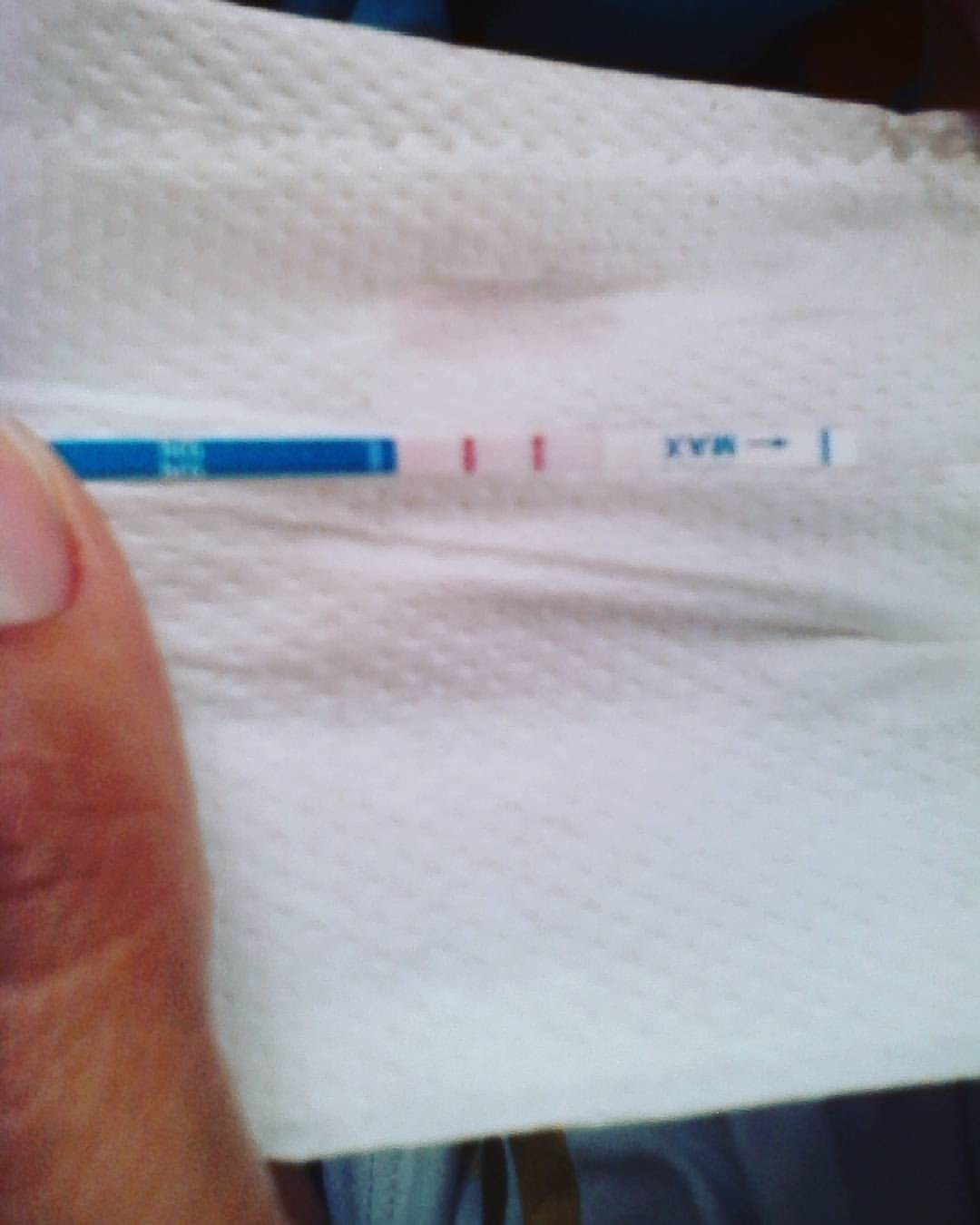This photograph captures an intimate and significant moment as a woman examines a positive pregnancy test. The close-up image focuses on her light-skinned hand, showcasing a neatly manicured thumb, which firmly grasps the test against a roll of toilet paper in the upper left-hand corner. The toilet paper’s surface reveals tiny white dots and ridges, characteristic of its texture. 

Prominent in the center is the pregnancy test stick, held upside down. The handle of the stick is a bright blue adorned with small white dots. Moving from left to right, the test displays a wet section where the chemical reaction occurs. This section reveals the decisive outcome—two red lines indicating a positive result.

In the bottom center to the bottom right corner, a splash of dark and light blues from an undefined background adds depth and contrast to the image. The test stick also bears the label "MAX" with a blue arrow pointing to the right, further emphasizing its orientation and authenticity. The emotions of anticipation and realization are palpable in this closely-cropped, declarative photograph.